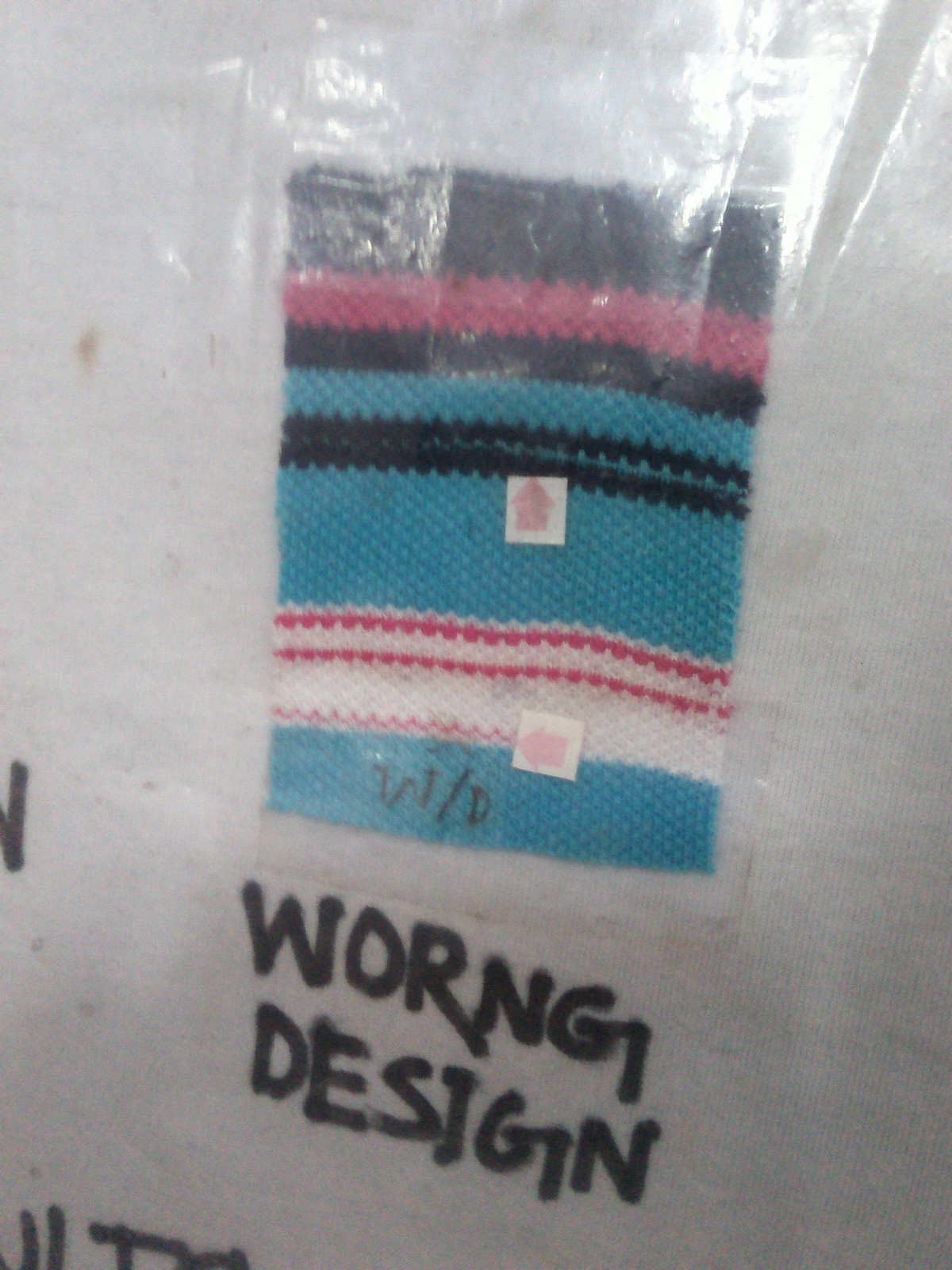The image depicts a close-up of a wristband sample taped onto a white background, likely a piece of cardboard or poster board. The wristband, encased in a glossy plastic bag, stands out prominently due to its colorful pattern and reflective surface. The design of the wristband comprises a series of color bands: starting from the top, there is a thick black line, followed by a thinner pink line, another black line, a thin turquoise line, and then a sequence of very thin black, blue, and black lines. Further down, there is a wide turquoise strip, a white line, a thin pink line, another white line, another thin pink line, a wider white line, a thin pink line, and finally a very thick blue line at the bottom, on which "W-D" is written in black marker. Beneath the wristband, in bold black print, the words "WONG DESIGN" are displayed, with the word "WONG" being misspelled as "W-O-R-N-G." The overall presentation suggests it is a sample of fabric design, highlighted by the repetitive use of colors and annotated labels, possibly pointing out errors or areas of note within the design.